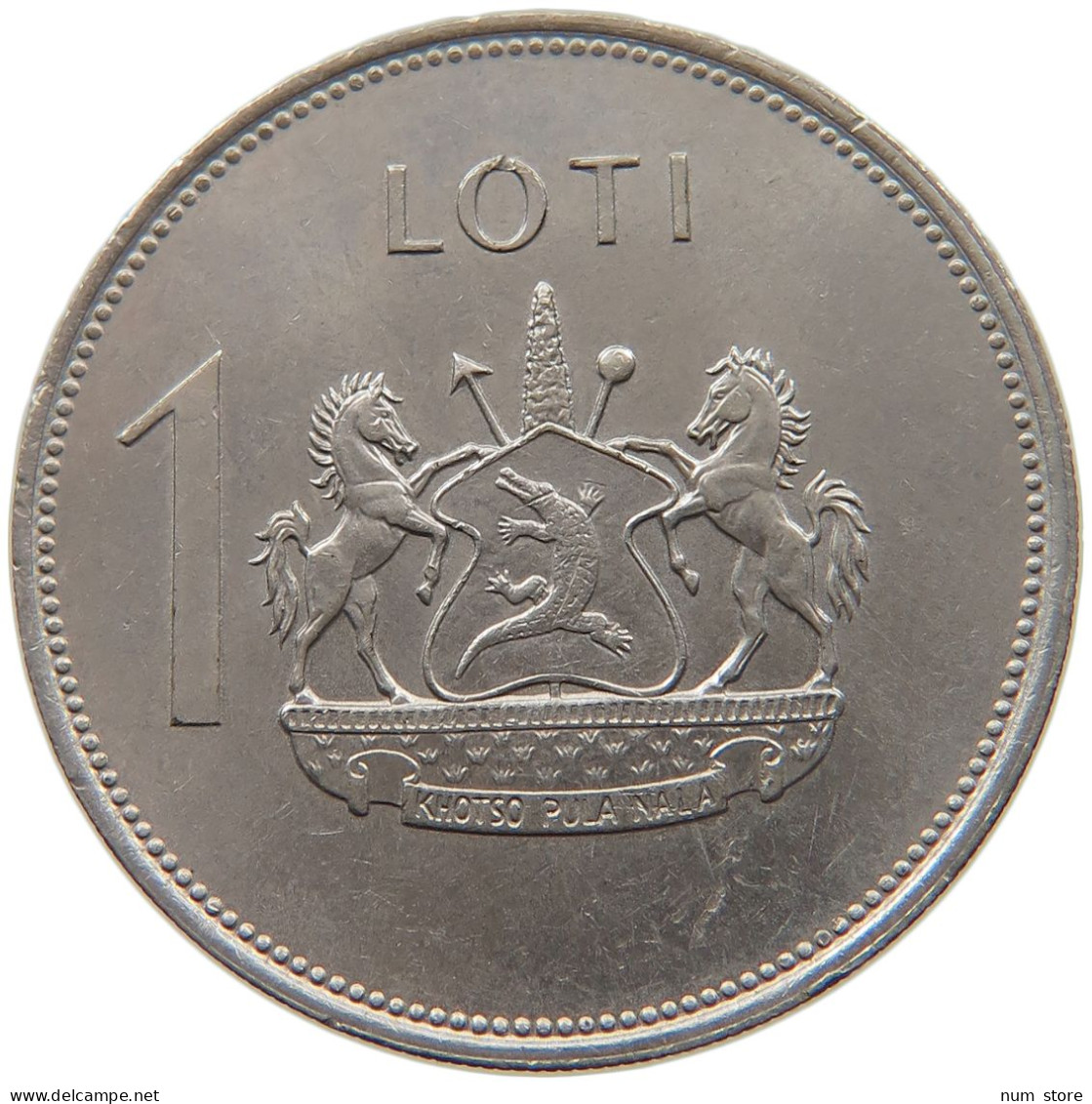This photograph captures a coin with intricate details. The coin, likely part of a promotional ad given the presence of URLs—www.delcampe.net in the lower-left corner and "numstore" in the bottom-right corner—is primarily silverish in color, although one description mentions it as being a dull copper. At the top of the coin, "L-O-T-I" is prominently engraved. To the left, there's a number "1." The centerpiece of the design features a heraldic emblem with two horses rearing up and facing each other, placing their forelegs on a central shield that depicts an alligator or crocodile. The shield is detailed with additional elements: arrows, circular shapes, and triangles. Beneath this heraldic image, there's an inscription that seems to read "Kotso Pula Nala," accompanied by a scroll or boat-shaped design with a grass-like pattern. The coin is depicted with high detail, making its exact size indeterminate.